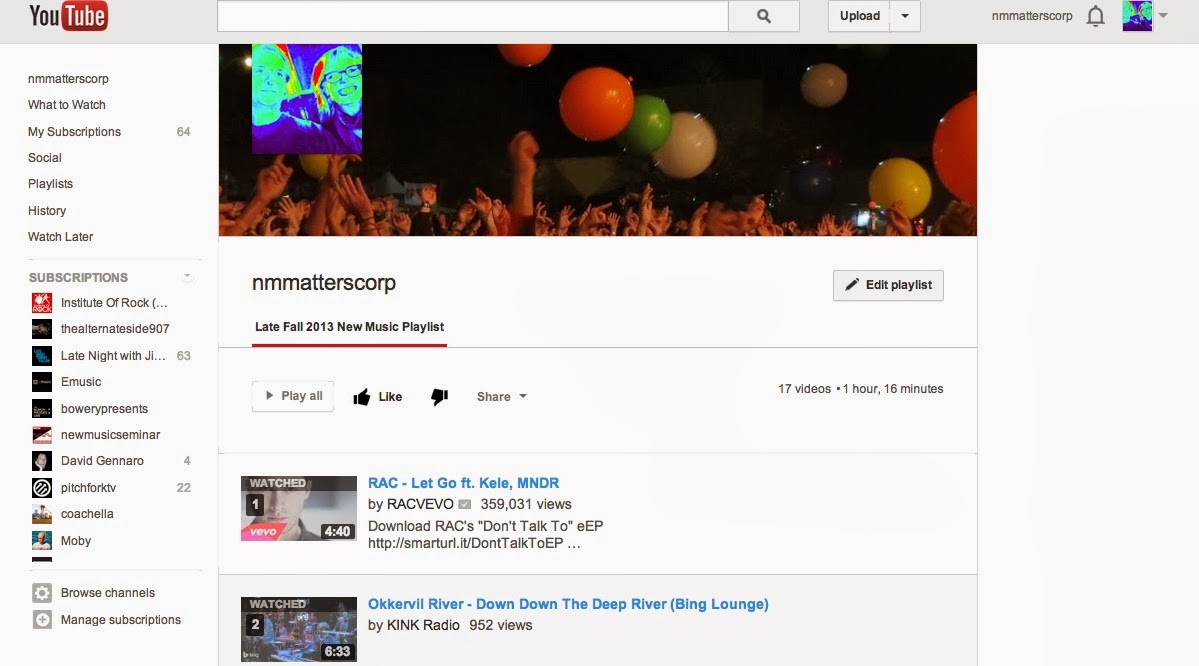Screenshot of the YouTube website interface:

In the upper left corner, the red YouTube logo is prominently displayed. Spanning across the top of the screen is a search bar with a magnifying glass icon at its end. Adjacent to the search bar is a box labeled "Upload". On the far right of the top bar, the user's account information is visible, showing the letters "N.M. Matters Corp.", followed by a bell notification icon and a profile picture that is a mix of green and blue, though the details are indistinguishable.

In the left-hand column of the page, the following menu options are listed:
- N.M. Matters Corp.
- What to Watch
- My Subscriptions (64)
- Social
- Playlists
- History
- Watch Later

Below these main categories, the word "Subscriptions" appears, under which several subscribed channels are listed, including:
- Institute of Rock
- The Alternate Side 907
- Late Night with Jay
- eMusic Bowery Presents
- New Music Seminar
- David Gennaro
- Pitchfork TV
- Coachella
- Moby
- Browse Channels
- Manage Subscriptions

In the central area of the screen, a large image depicts a lively outdoor celebration with people raising their arms and colorful balloons floating in the air. Below this image, text reads:
- N.M. Matters Corp.
- Edit Playlist
- Late Fall 2013
- New Music Playlist

Options under the playlist include:
- Play All
- Thumbs up icon with the word "like"
- Thumbs down icon
- The word "Share"

Additionally, the playlist details note that it contains 17 videos with a total runtime of 1 hour and 16 minutes.